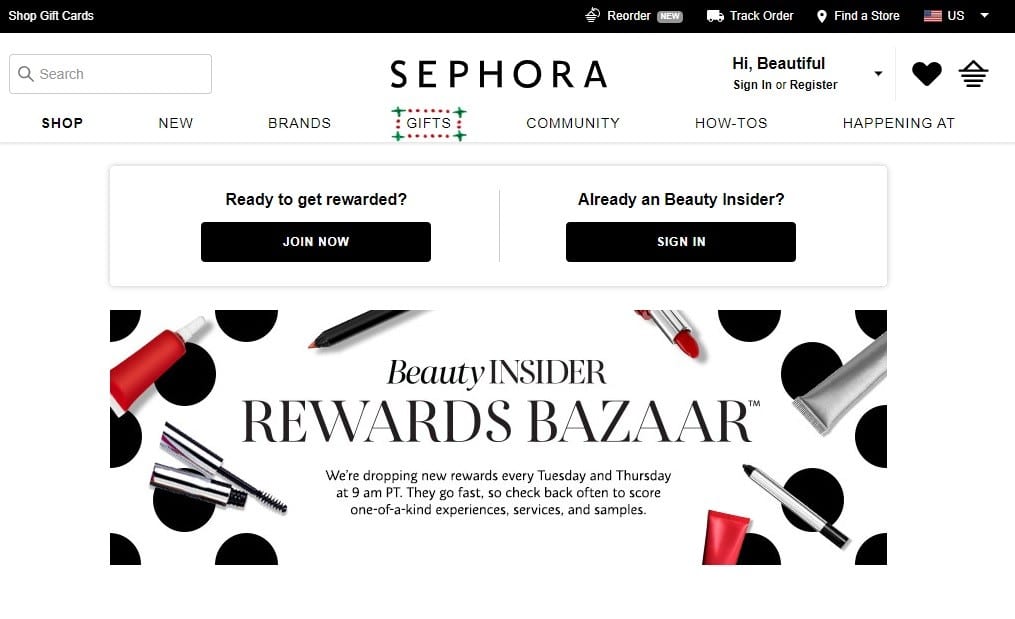The website image displays a well-organized layout with various sections and features highlighted. At the very top, there is a sleek black banner. On the left side of this banner, the text "Shop Gift Cards" is displayed in white with capitalized initials (S, G, C). Moving towards the right, there is a "Reorder" option. Further right, a small, rounded rectangle features the word "NEW" in capital letters, adjacent to a truck icon labeled "Track Order." Continuing to the right, there's a location marker labeled "Find a Store" and a U.S. flag accompanied by a “U.S.” drop-down menu.

Below the black banner, the background shifts to white. On the left hand side, there is a search bar with a magnifying glass icon and the word "Search" inside. Centrally positioned is the brand name "SEPHORA" in bold, capital letters. Directly to the right, it says "Hi Beautiful! Sign In or Register," followed by a drop-down menu, a black heart icon, and a black-and-white shopping bag icon.

Further down, there is a navigation menu with categories listed from left to right: "Shop" (in darker text), "New," "Brands," "Gifts" (marked by a square decorated with red and green dots arranged at the corners), "Community," "How-To's," and "Happening At."

Moving down the page, another section invites users to "Ready to Get Rewards? Join Now" and indicates "Already a Beauty Insider? Sign In." Below this is a prominent banner image for the "Beauty Insider Rewards Bazaar." This banner is adorned with small black dots at the corners and features pieces of makeup products. Text on the banner announces: "We’re dropping new rewards every Tuesday and Thursday at 9 a.m. PT. They go fast so check back often to score one-of-a-kind experiences, services, and samples."